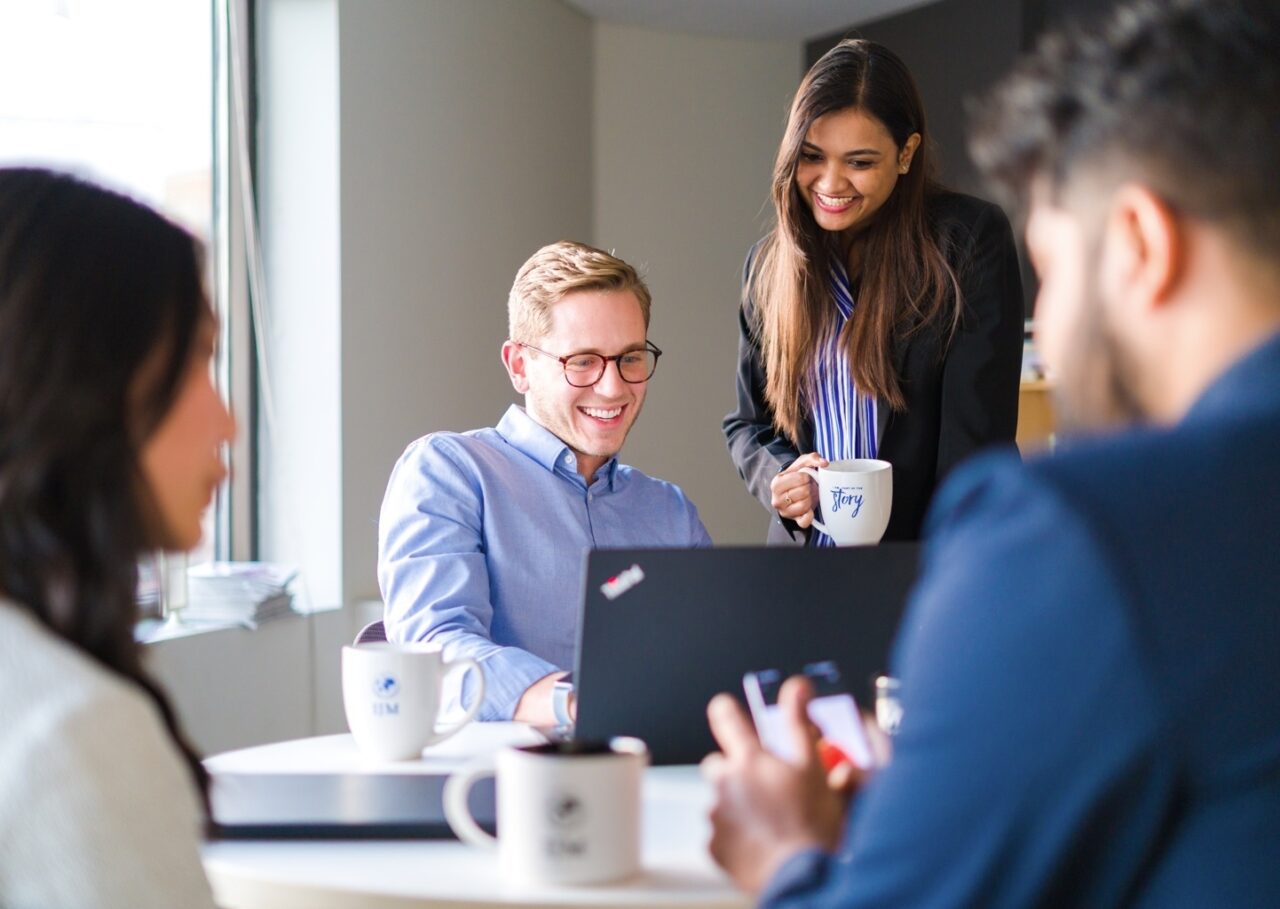In an office setting, a man and woman stand prominently in front of a black laptop, both smiling as they engage with its screen. The man, with fair skin, blonde hair, and brown round-shaped glasses, wears a blue button-up shirt. His female colleague, who has light brown skin, long dark brown hair, and red lips, is dressed in a black suit jacket over a blue and white striped undershirt. She holds a white mug featuring blue text. The foreground is slightly blurred, showing two additional individuals: a man in a blue suit jacket and a woman in a white long-sleeve shirt, both looking at a cell phone on a white circular table. Surrounding them are more white mugs, some inscribed with words. A folded laptop lies nearby, and to the left, sunlight filters through a window, illuminating the scene framed by plain white walls.